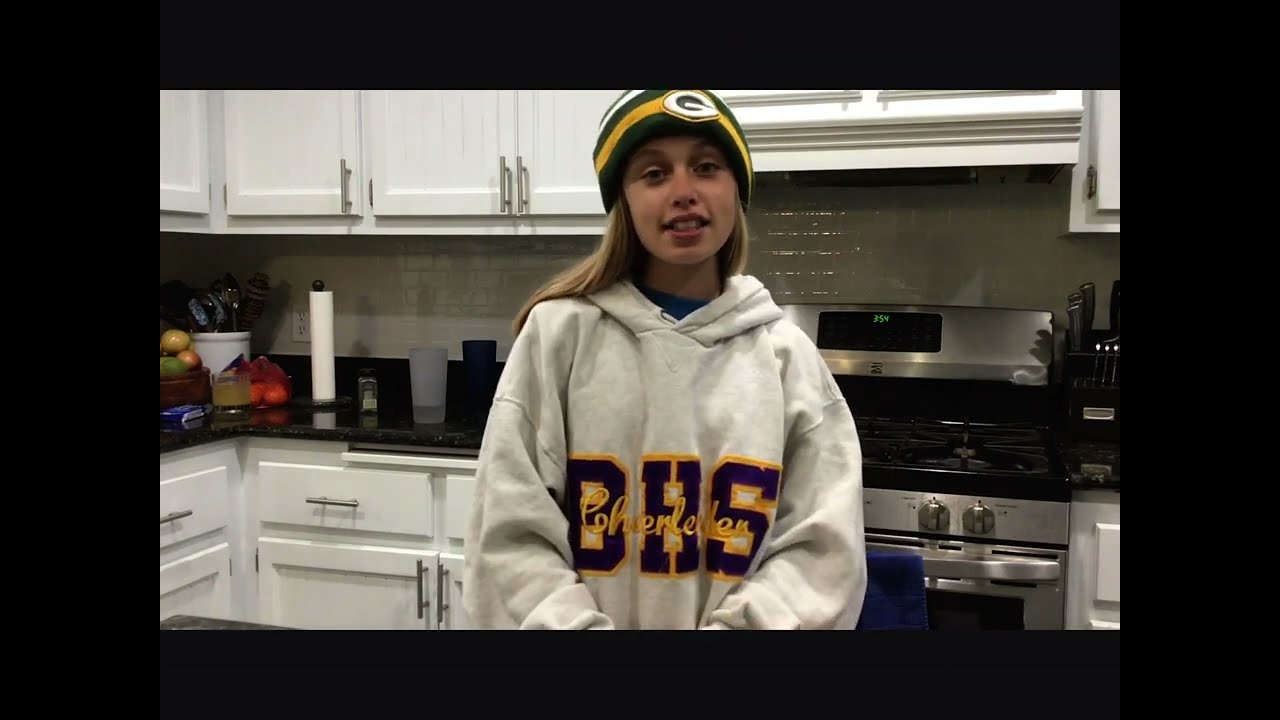In the center of the image is a young girl, likely a teenager, clad in a light gray BHS cheerleading hoodie, prominently displaying dark letters with yellow cursive embroidery overlaid. She also dons a Green Bay Packers beanie adorned with dark green, yellow, and white stripes and a central "G" emblem. Her long, blonde hair is draped behind her back, and she appears to be looking at something off to the side, possibly speaking.

The backdrop is a well-equipped kitchen featuring white upper and lower cabinets with sleek silver handles. The countertops are a sophisticated mix of black and white marble. To the right, there is a stainless steel oven and range, and a set of stainless steel knives in a black butcher block. The countertop also holds a paper towel roll, a glass with a clear liquid, and a collection of fruits and vegetables, including oranges. On the left side, additional items such as a bowl of fruit and a round ceramic container filled with various cooking utensils can be seen, completing the detailed and bustling kitchen environment. The image is framed by thick black borders on the sides and thinner black borders on the top and bottom.